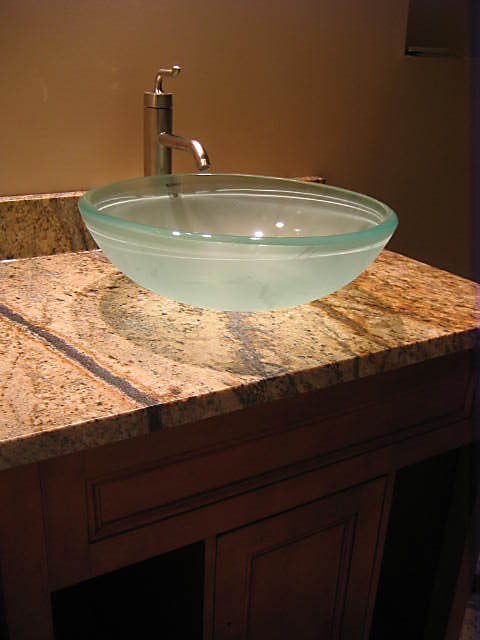This image showcases a sophisticated and modern sink setup. The countertop is made of light brownish granite with intricate patterns, featuring a small, 2-inch tall backsplash. Below the countertop, there's a wooden cabinet with a light wood grain finish and dark accents, adding a touch of elegance. The photograph is taken from an angle that reveals both the surface of the countertop and part of the storage space underneath.

The centerpiece of the setup is a bowl-shaped sink, made from a clear yet slightly frosted material, lending it a delicate, ethereal appearance. The rim of the sink is transparently defined, giving it a refined edge. Complementing the sink is a faucet designed to mimic an old-fashioned water pump, characterized by a tall cylindrical base and a curved spout that directs water straight into the sink.

The background wall is painted in a light tan color, transitioning into a darker shade towards the right of the image, creating a gentle gradient effect. In the upper right corner, there's a blacked-out window, possibly hinting at either nighttime or some form of shading. Underneath the countertop, the open cabinet doors reveal dark, empty spaces, adding depth to the image.

An artistic dark stripe on the granite runs to the left of the sink, extending to the front edge of the countertop and highlighting the seamless transition between the granite surface and the wooden cabinetry below. This blend of textures and details provides a striking visual contrast, enhancing the overall modern and stylish aesthetic of the space.